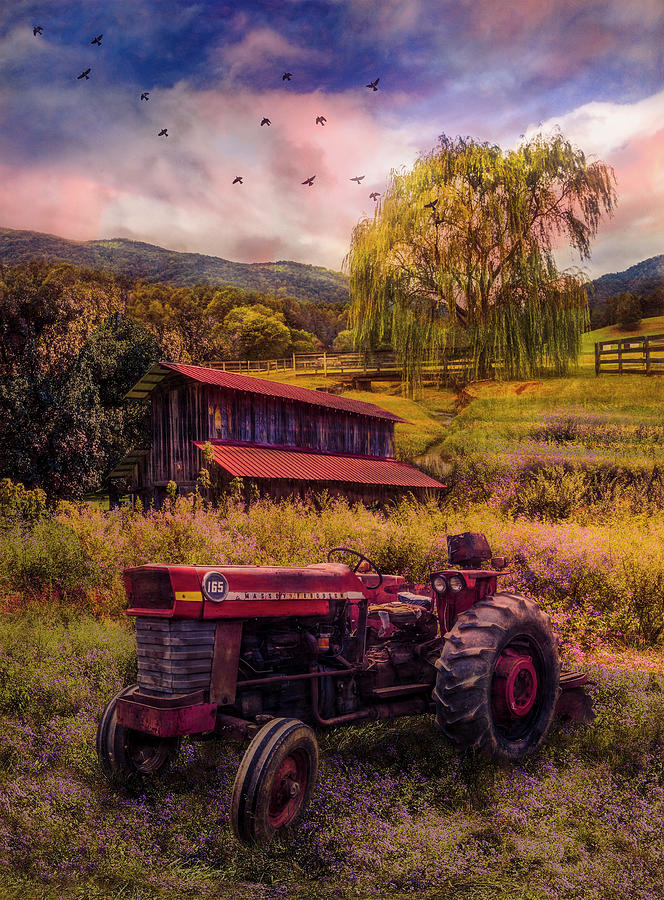This is a color photograph that captures a picturesque yet slightly surreal farm scene. In the foreground, an old, rusted red tractor with the number 165 painted in white on its side rests idly in a slightly overgrown field. Its front wheel is smaller than the back, and both appear worn and dilapidated. To the left stands a red barn, equally aged with a matching red roof. The vast expanse of sky above features a blending palette of blue, pink, and white hues, dotted with dark birds flying across. This sky's almost artificial look suggests possible photo adjustments. In the background, rolling green hills are visible, encircled by a white fence. To the right, a grand weeping willow tree with yellowish-green, drooping leaves adds a touch of natural elegance to the scene.